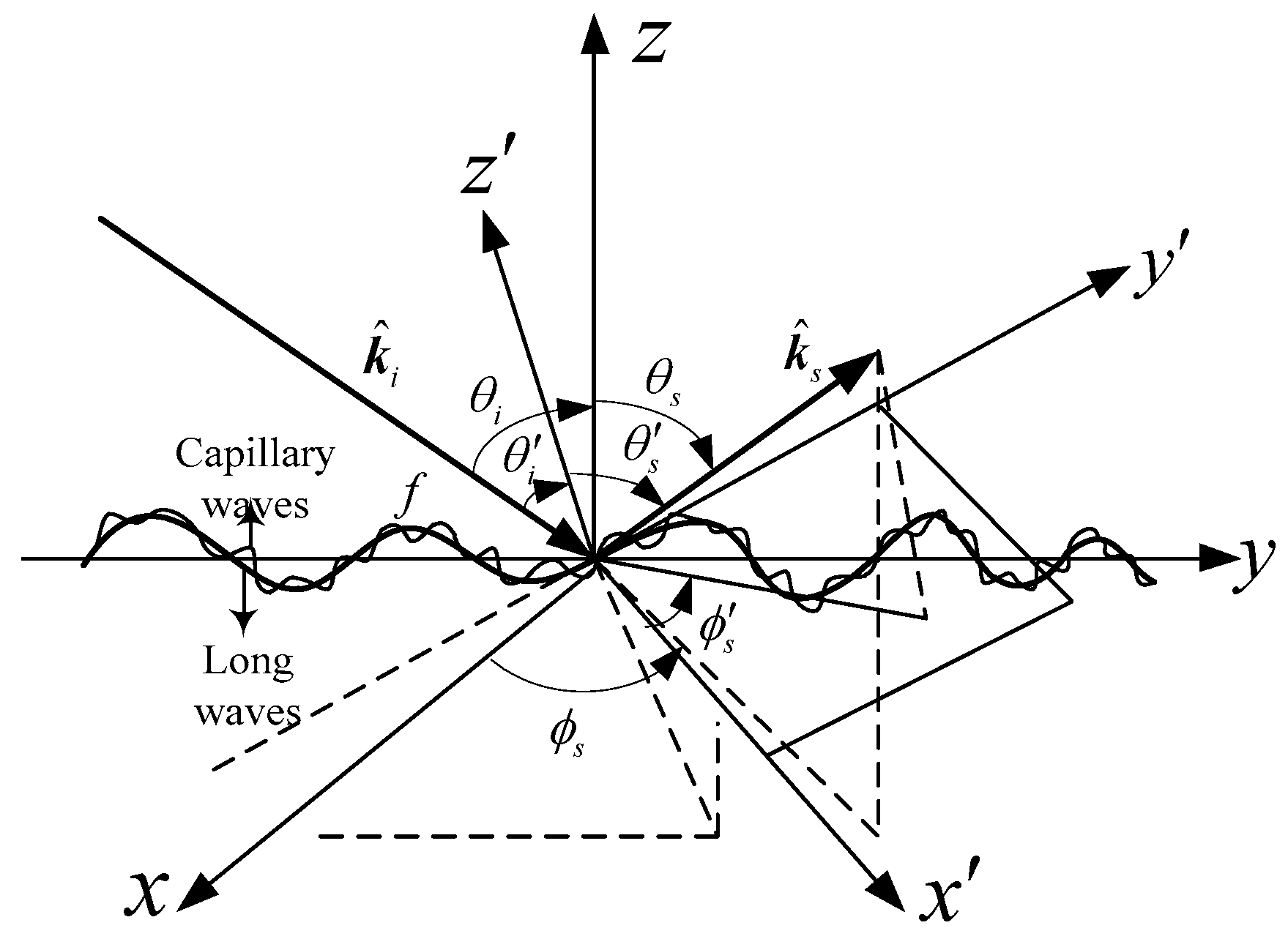This black and white illustration depicts a detailed scientific chart on a white background. Central to the image are numerous black lines radiating from a central point, varied in style and thickness; some lines are solid, others are dashed, and some end with arrowheads. These lines include labels such as X, X', Y, Y', Z, Z', Kᵢ, and Kₛ. Notably, a wavy line runs centrally across the chart, with a smaller high-frequency wave superimposed upon it, possibly indicating wave phenomena.

Text is interspersed among the lines, with the notable terms "capillary waves" and "long waves" appearing on the left side of the illustration. Greek letters, including θ (theta) and κ (kappa), are also visible, suggesting the chart relates to physical sciences or physics. Additionally, dashed lines form right angles throughout, contributing to the overall structure of this complex diagram.